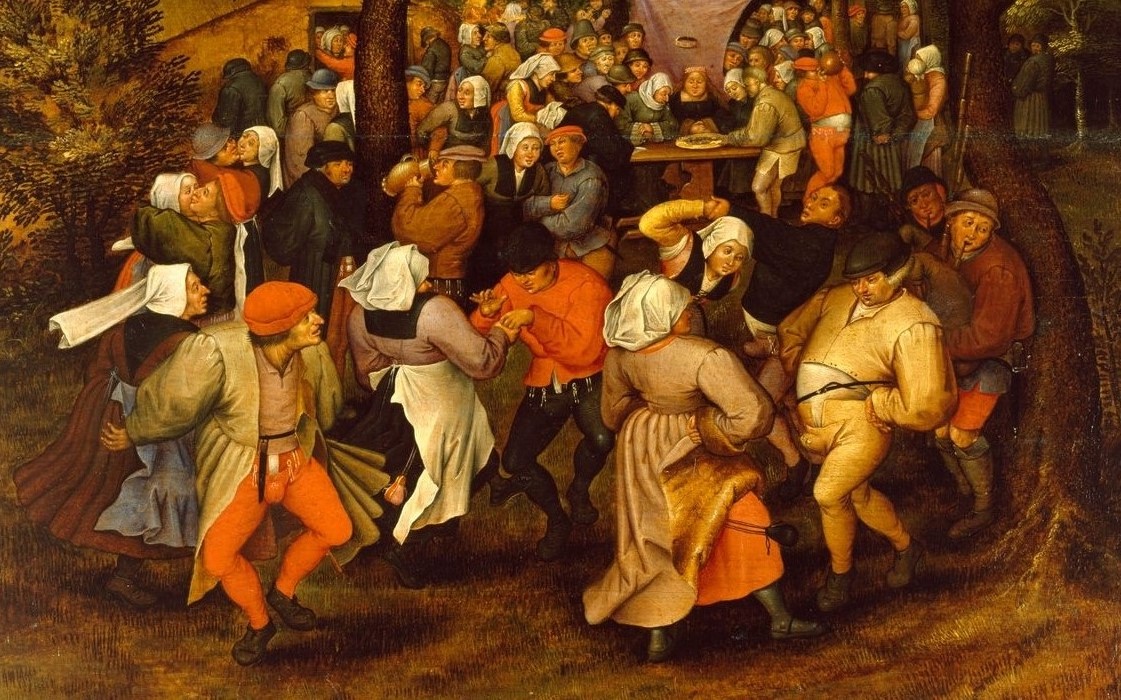The painting "Peasant Wedding Dance," created in 1604 by Peter Bruegel the Younger, captures a lively scene of rural 17th-century life during a wedding celebration. A multitude of peasants are depicted enjoying the festivities, characterized by their animated dancing and social interactions. Men are seen wearing tight-fitting pants with distinctive pouches at the groin, typical of the period’s fashion, paired with leather vests. Women are adorned with white scarves on their heads, and some couples are shown embracing intimately around the scene. Various elements add to the vibrant atmosphere: a man playing bagpipes, tables filled with revelers eating and drinking from large pitchers and jugs, and figures huddling in groups, suggesting an outdoor setting under scattered trees. The earthy color palette of browns, oranges, and tans brings a rustic vibrancy to the scene. Hanging in a museum, this oil painting offers a detailed glimpse into the joyful and communal aspects of peasant life during the Renaissance.